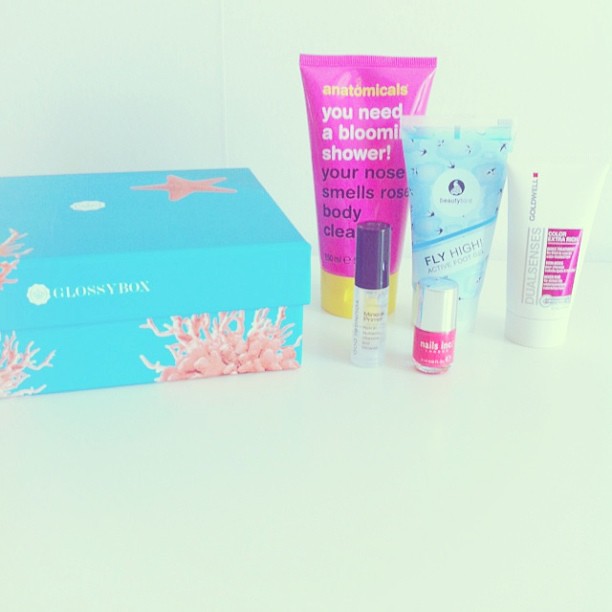The image features an array of personal care products displayed against a very light blue, almost white, faded background. Dominating the left side is a bright aqua-blue box adorned with pink coral and starfish motifs. The box prominently displays the brand name "Glossy Box" in white text. 

To the right of this box, a collection of five different items is neatly arranged. At the forefront is a pink tube with a yellow cap, bearing the text "Anatomicals. You need a blooming shower. Your nose smells rose," indicating it's a body cleanser. There is also a tiny clear glass bottle with a black cap next to a miniature pink nail polish sample bottle, half its height and with a silver cap, labeled "Nails."

Behind these small items are three tubes. The first is a large pink tube with text running vertically, reading "Anatomicals." To its right, a very light blue and white tube titled "Fly High" features black bird outlines, suggesting it is an active foot gel. The final item, a white tube with a pink label and tiny white letters, reads "Dual Sense," although its purpose isn't clear. All products rest on a pristine white table surface, contributing to the clean and fresh aesthetic of the image.